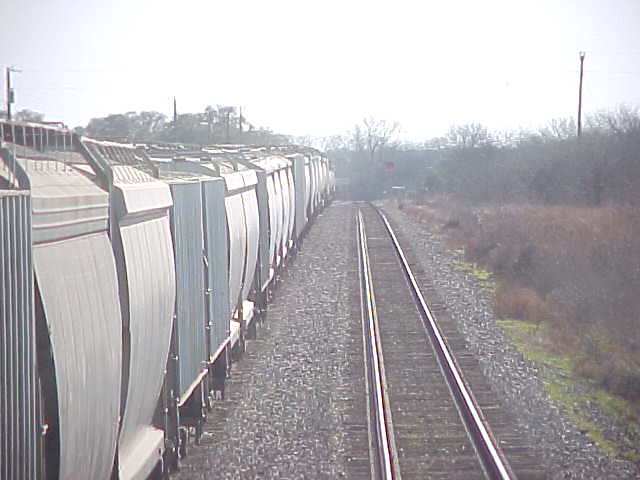This photograph captures two parallel sets of railroad tracks stretching into a wooded area, disappearing into a horizon lined with leafless trees and brown bushes. The viewpoint is slightly off-center and elevated, providing a clear, detailed view of the scene. On the left track, a stationary train extends into the distance with boxcars in various shades of gray, silver, blue, and possibly dark hues, though the exact colors are difficult to discern due to slight overexposure. The right track is empty, flanked by gray and white gravel that transitions into patches of green grass and scraggly brown brush. The sky is a uniform white, suggesting cloud coverage with a bright light source, possibly the sun, creating a noticeable lens flare near the tree line. Additionally, there are light posts or electrical poles visible in the background, as well as a train crossing and warning light further enhancing the depth and realism of the scene.